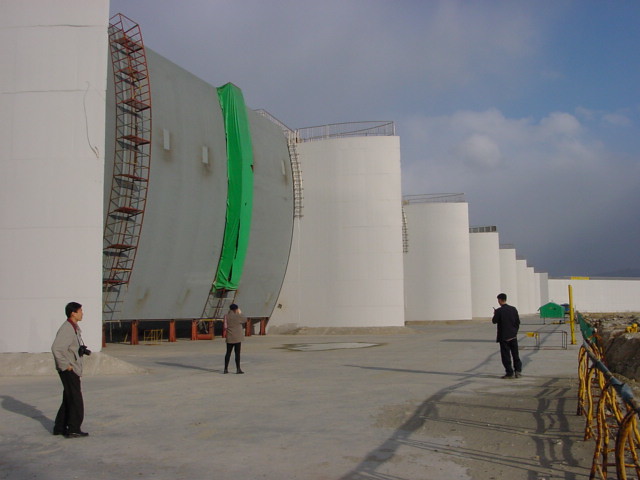The photograph depicts a vast engineering project, likely related to flood control or dam infrastructure. Along the left side of the image, a series of tall structures resembling fins, covered in white material and topped with metal railings, dominate the view. Between two of these fins in the foreground, a large convex structure stands out, equipped with a red metal ladder and platforms climbing up its left side—suggesting it functions as a gate mechanism. 

In the lower section, a grey tarmac or concrete pathway extends into the distance on the right-hand side. Three individuals are visible: a man on the left wearing a green windbreaker, black pants, and black shoes, with a large camera around his neck, possibly of Asian descent; a woman to his left, seemingly raising her hands to her face as if taking a photograph; and another man dressed head-to-toe in black, holding a walkie-talkie, positioned towards the right. The background sky is predominantly cloudy with whitish-grey tones, but a patch of blue sky peeks through in the top right corner. There is also a green tarp over one of the structures, adding a splash of color to the otherwise industrial scene.